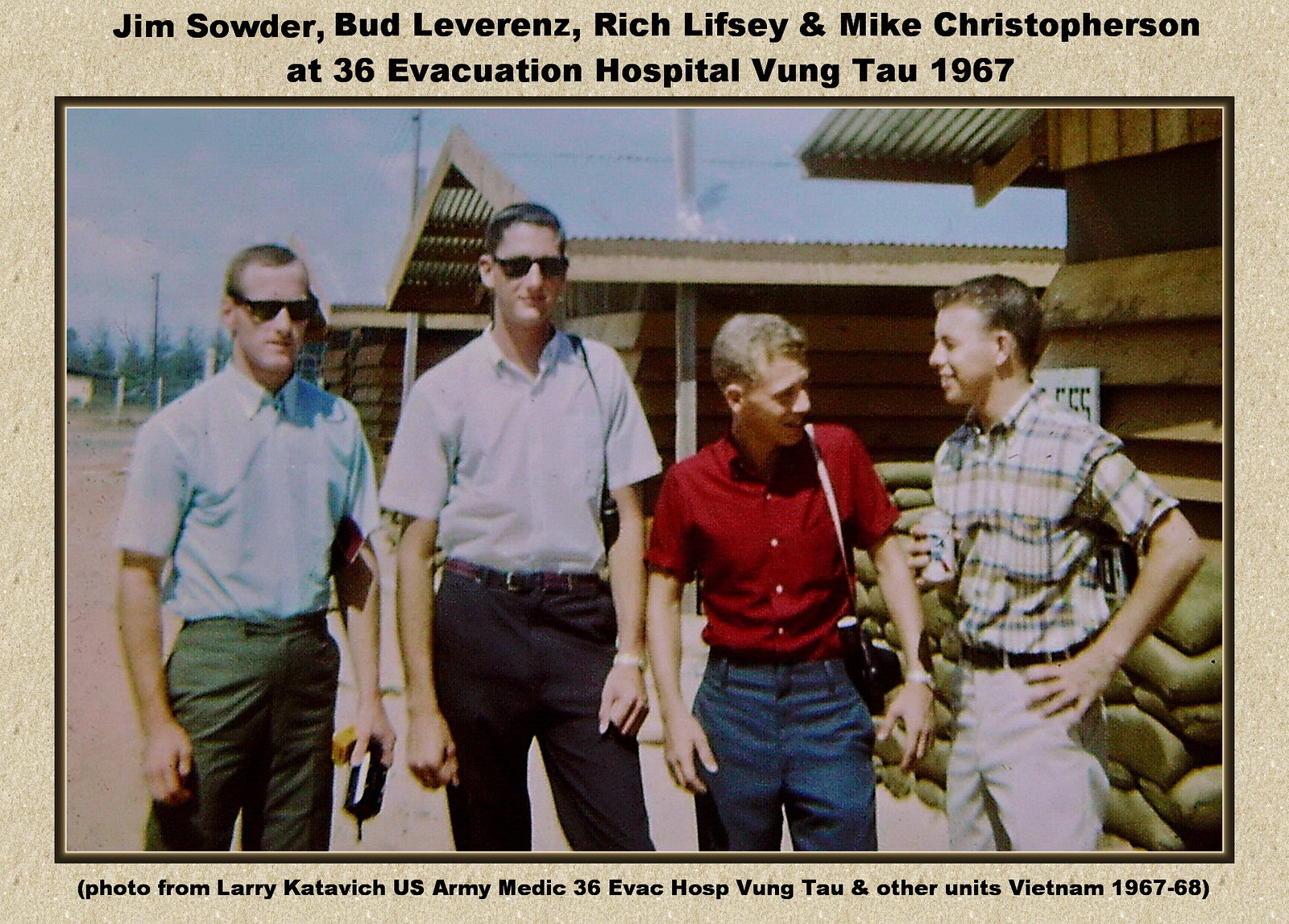This photograph captures a moment shared by four young men at the 36 Evacuation Hospital in Vung Tau, 1967. The two individuals on the left are facing the camera, while the two on the right are engaged in conversation with each other. 

The first man on the left is sporting a light blue button-up collared short-sleeve shirt paired with greenish-gray pants. He wears sunglasses and has very short hair. Standing next to him, the second man also has short hair and sunglasses. His outfit consists of a white top and blue pants.

The third man, who is turned towards the fourth, has light brown hair and is dressed in a red shirt and blue pants. The final individual in the group wears a plaid shirt and khaki pants. Both of these men are smiling as they converse with each other.

In the background, sandbags and several buildings with metal roofs are visible. These structures appear to serve temporary purposes and are not residential homes or simple sheds, but rather sturdier constructions likely put up for utilitarian needs.

The photograph is bordered in brown, with text at the top identifying the men as Jim Souder, Bud Leverenz, Rich Lifsey, and Mike Christofferson at the 36 Evacuation Hospital, Vung Tau, 1967. Below this is another line of text in parentheses: “photo from Larry Katowicz, U.S. Army medic, 36 Evac Hospital, Vung Tau, and other units, Vietnam, 1967-68.” The sky in the background is clear and blue, providing a serene backdrop to this historic moment.